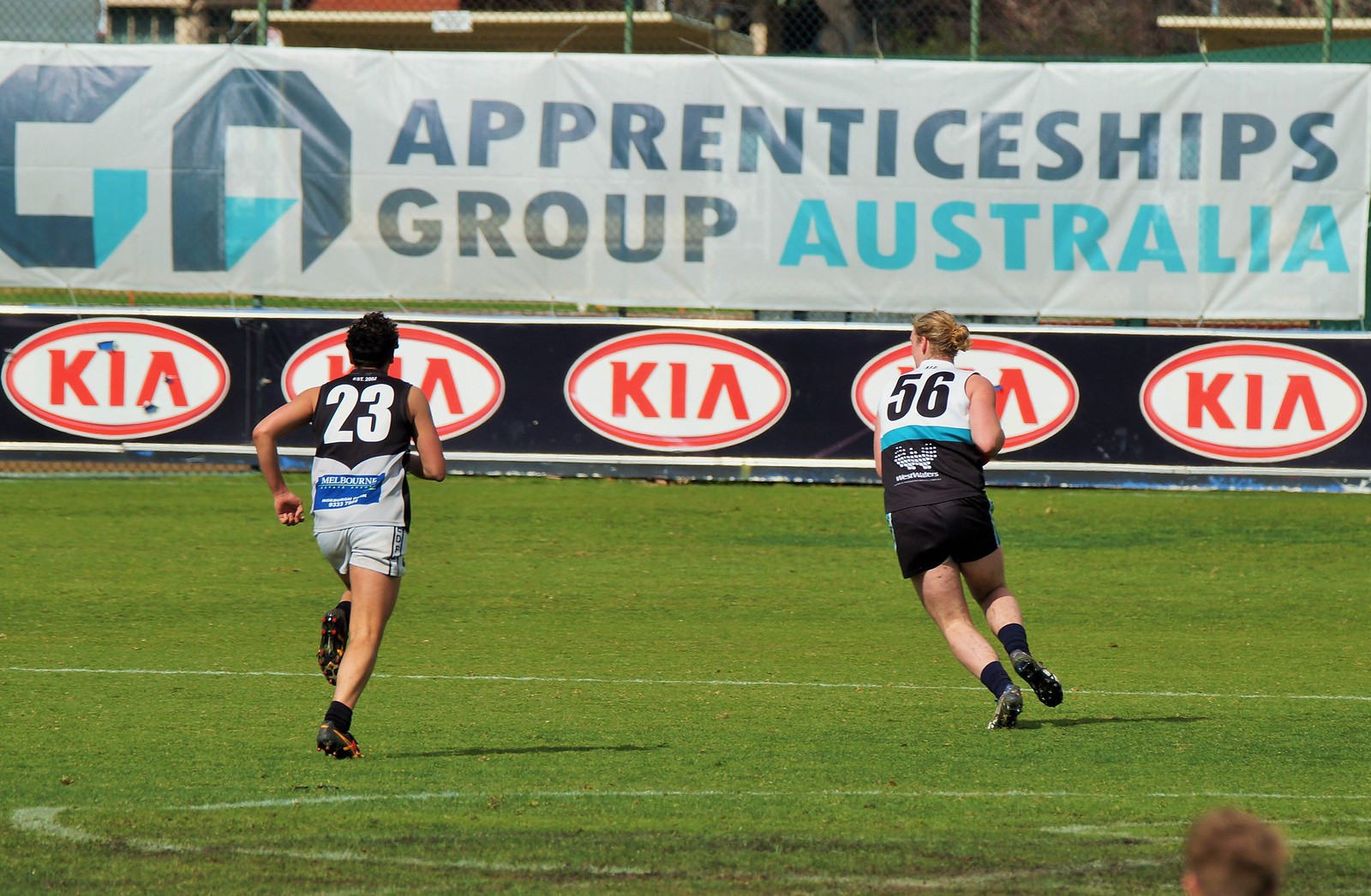The image captures an outdoor soccer match on a sunny day, featuring two male soccer players sprinting across a grassy field lined with white chalk markings. The player on the left, with short dark hair, is dressed in a black and gray uniform, numbered 23. The player on the right, with blonde hair tied back, sports a white, teal, and black uniform, numbered 56. In the background, a large banner runs along the sideline of the soccer field. This banner prominently displays "Apprenticeships Group Australia," with the word "Australia" in blue font and a grey and blue "GA" logo on the left-hand side. The bottom of the banner is black, featuring the red Kia logo repeatedly printed across it. Additionally, there are spectators or additional players visible in the foreground.